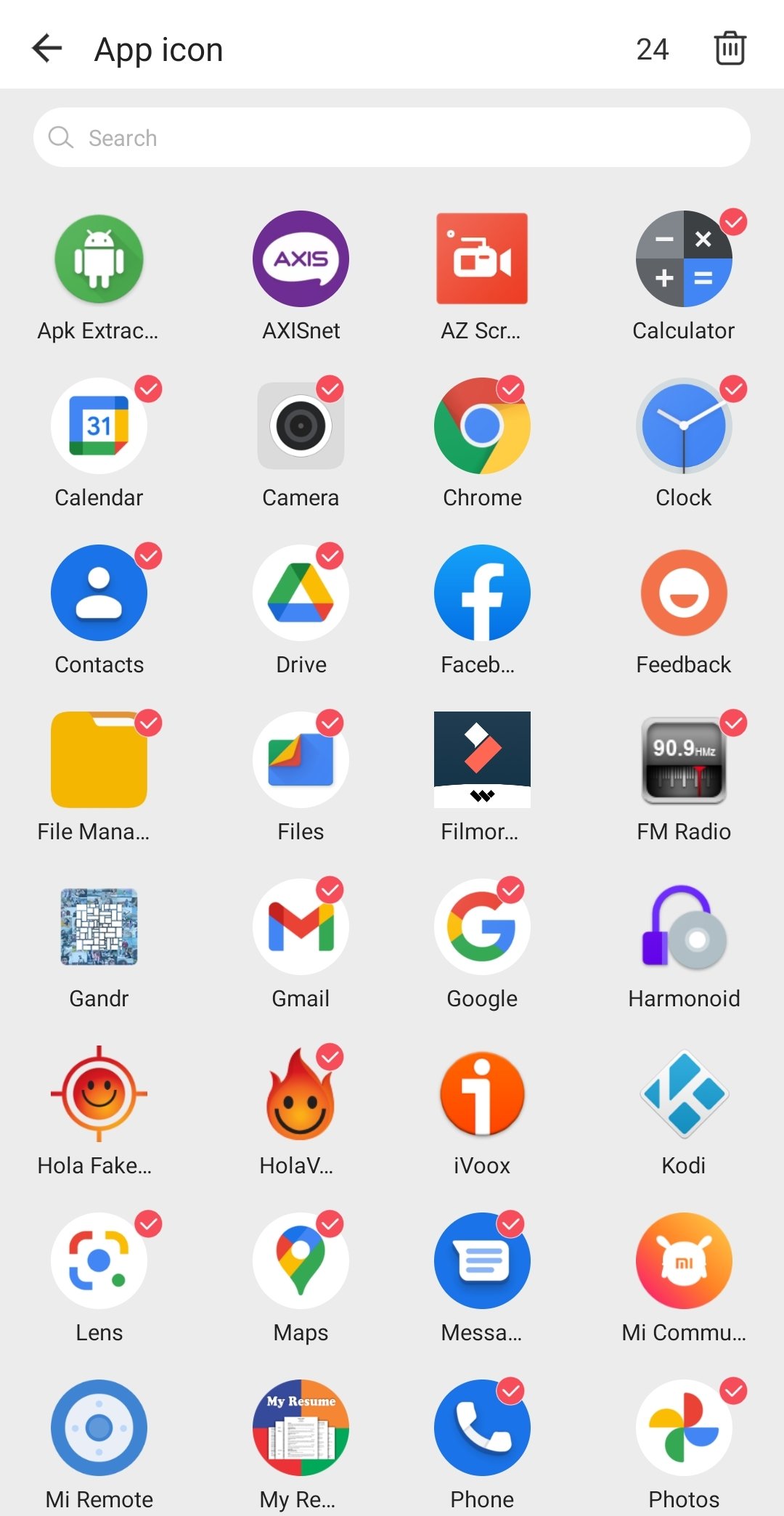This screenshot appears to be taken from a mobile phone, featuring what looks like an app management interface. The interface might be part of a customized app drawer or a specific application designed for organizing apps. 

In the top-left corner of the screenshot, there is a black arrow pointing to the left, followed by the text "App Icon." On the top-right corner, the number "24" is displayed next to a trash can symbol, likely indicating a total of 24 app icons present on this screen. Below this top bar is a search box, useful for quickly finding specific apps.

The main section of the screenshot displays 24 app icons in a grid format. Several of these apps, such as Google Photos, Google Lens, Google Maps, Google Messages, Phone, Gmail, Google Search, Google Files, Google Contacts, Google Drive, Google Chrome, Google Calendar, Calculator, Clock, and Facebook, are easily identifiable. Some of these app icons feature a small red circle with a white check mark in the upper right corner, signifying that these apps have been selected by the user.

The detailed arrangement and labeling within the interface suggest a highly organized and user-friendly environment, providing an efficient way to manage, search, and select multiple applications at once.